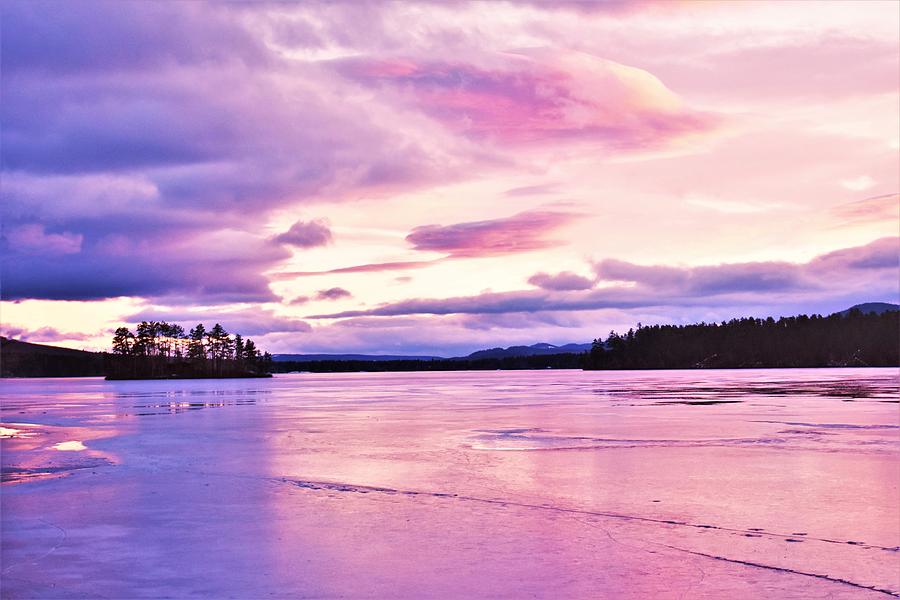This landscape photograph captures a serene, vibrant scene during either sunrise or sunset, casting a predominantly purple and pink hue across the entire image. In the foreground, a wide body of water showcases gentle ripples tinged with these hues, hinting at a partially frozen surface with visible ice in places. The horizon cuts across the middle of the photograph, marking the meeting point of the water and the sky. 

On the horizon's right side, the silhouette of many trees stands out against the colorful sky. To the left center, a small island dotted with numerous pine trees is visible. The left side of the image features a gradually rising hill, giving depth to the landscape. The sky, laden with light blue and white clouds, transitions into a blend of white, yellow, pink, and purple, beautifully reflecting the sunlight. Heavy cloud coverage in the upper part of the picture picks up these colors, adding to the ethereal atmosphere of this tranquil scene.